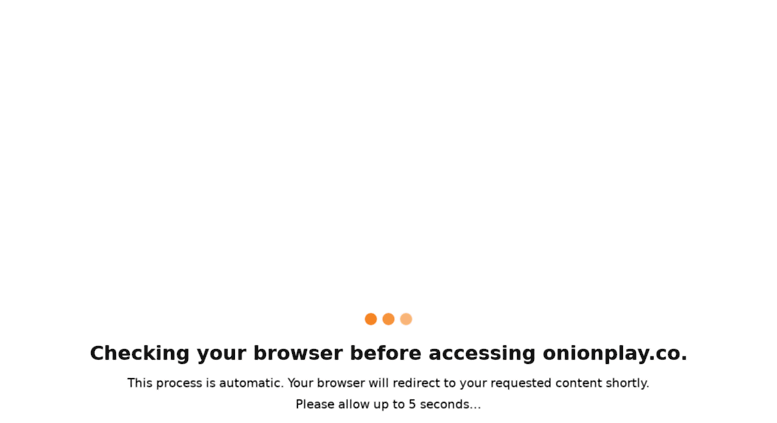The image is a rectangular screenshot of a browser page, illustrating an interstitial page typically seen while information is being submitted. Occupying the bottom 15-20% of the image is a centered notification section against a white background. The notification features bolded, large black text reading, "Checking your browser before accessing onionplay.co." Beneath this primary message is a smaller-font note stating, "This process is automatic. Your browser will redirect to your requested content shortly. Please allow up to five seconds..."

Above this text is a horizontal arrangement of three orange dots: the leftmost dot is a darker orange, the middle dot is a standard orange, and the rightmost dot is a lighter orange. The vast majority of the image, primarily the top portion, is a plain white space, suggesting that the screenshot was likely taken midway through the browser's verification process, capturing just the bottom segment where the message and dots appear.